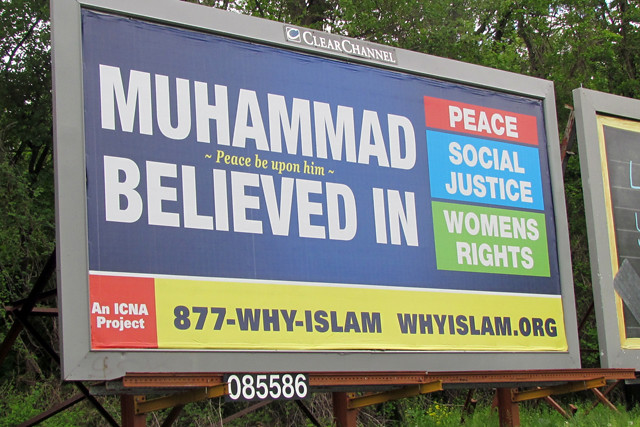This image features a prominent rectangular billboard erected on a heavily rusted metal scaffold. The billboard itself has a medium blue background and bears a powerful message in bold white capital letters: "Muhammad believed in." To the right, a red block containing the word "Peace" written in white letters stands out. Below this, the billboard highlights two more principles: "Social Justice" on a blue background and "Women's Rights" on a green background. 

Between the words "Muhammad" and "believed in," there are thin yellow letters with the phrase "Peace be upon him." At the bottom of the billboard, a banner with a red tip announces that this is "an ICNA project." Adjacent to this, a yellow banner displays the phone number "877-Y-Islam" in blue and the website "YIslam.org." Additionally, a small sign at the bottom of the billboard, set against a black background, shows a white numbering "085586." Only a small portion of a neighboring billboard is visible, hinting at its presence but not revealing its content.